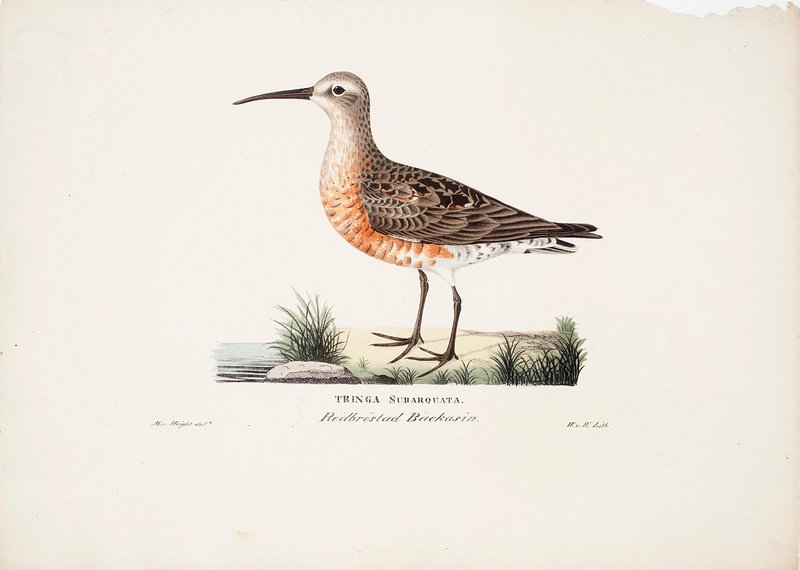This is a detailed pencil drawing of a medium-sized bird, approximately the size of a crow, identified as Tringa subarquata or "red-breasted bacchicin." The bird, depicted standing near the shore of a pond or lake, features a variety of distinct colors and markings. Its long, narrow beak and oval-shaped eyes accent its scientific illustration style. The bird has a tan head and back of the neck, with the front of the neck and chest showcasing lighter colors interspersed with orangish specks. Its underbody transitions to a deep orange and then back to white, decorated with brown polka dots as it moves towards the wings, which are brown with additional orange specks. The tail is primarily white with similar brown polka dots. The background of the drawing has a soft, very soft pink color, with minor water damage visible in the right-hand corner and at the top. The setting includes grass and water at the bottom, enriching the visual context of the bird in its natural habitat.